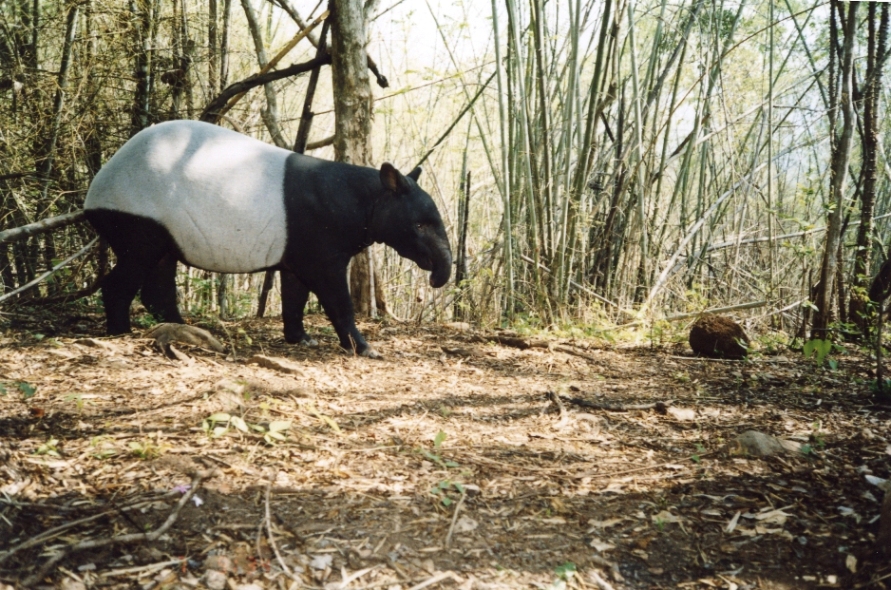This outdoor, daytime photograph captures a detailed scene dominated by a Malaysian tapir standing amidst a lush, wooded area. The sky above is a vibrant blue, with sunlight filtering through the thick canopy of tall trees, casting intricate shadows on the ground. The tapir, a large, unique animal with a small trunk resembling a baby elephant, has a striking appearance: its front half is black, while its middle to back, including its back legs, sport a prominent white patch, somewhat akin to a panda's coloration. Situated slightly left of center, the tapir seems to be gazing at a large brown rock on the right-hand side. Surrounding the animal are scattered dried leaves, weeds growing through them, and a wooden fence in the background, partially obscured by the forest foliage. The area also features bamboo plants, adding to the dense, wild setting.